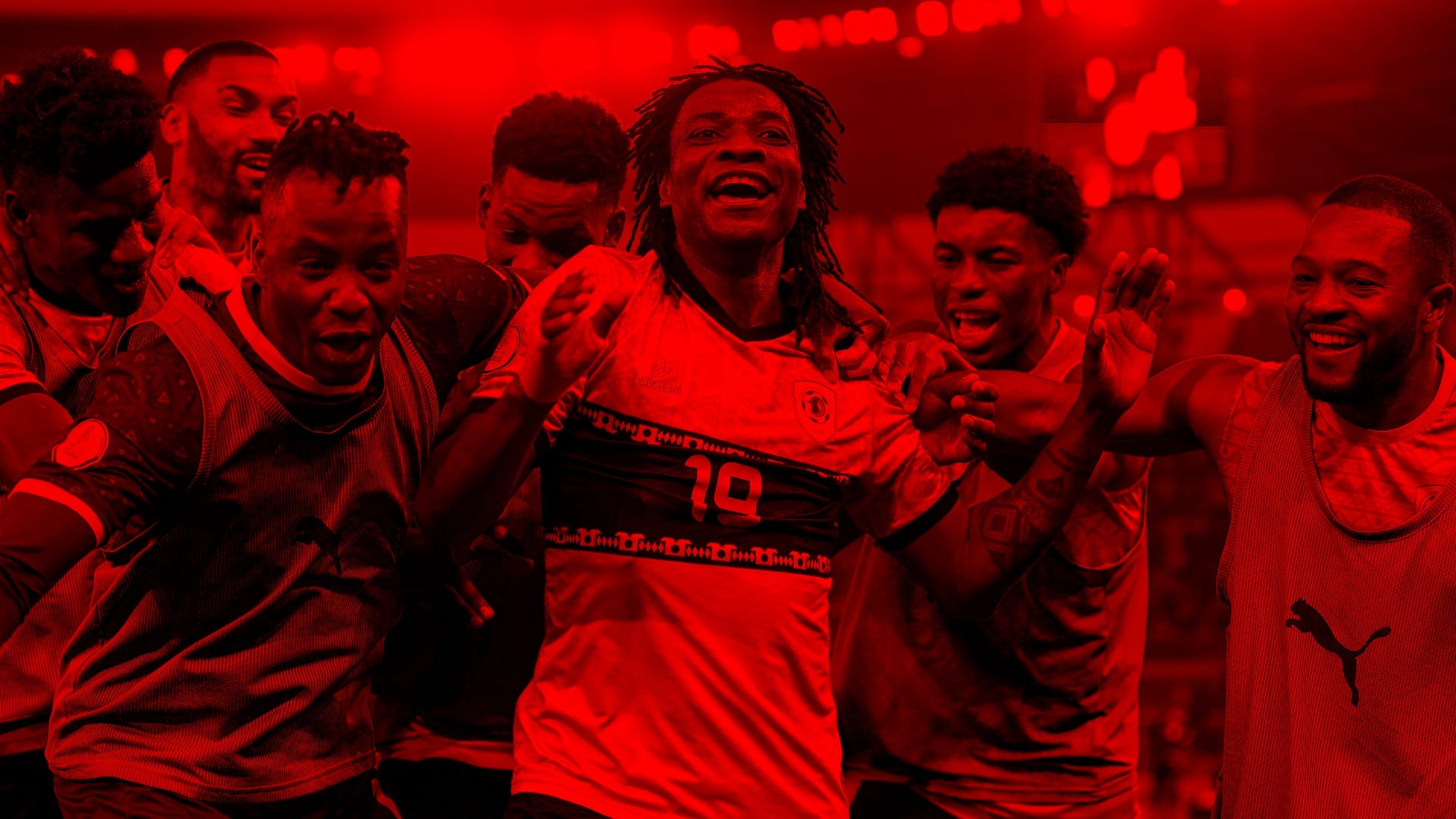This image showcases a jubilant moment featuring a group of six athletes, likely a soccer team, celebrating a victory. The entire scene is enveloped in a vivid red hue, casting a bright red tint over everything due to the lighting. At the forefront, a player donning a jersey with the number 10 raises both hands in triumph while smiling and looking upwards. He sports dreadlocks or braids and tattoos on his left arm. Surrounding him are five other players, who also seem to be in high spirits. Mixed in their attire are Puma T-shirts and jerseys similar to the central figure's. The players exhibit diverse hairstyles, including long hair, very short hair, and afros. In the background, there appears to be a scoreboard, and hints of an arena with spectators seated in bleachers, although these details are obscured by the pervasive red tint.